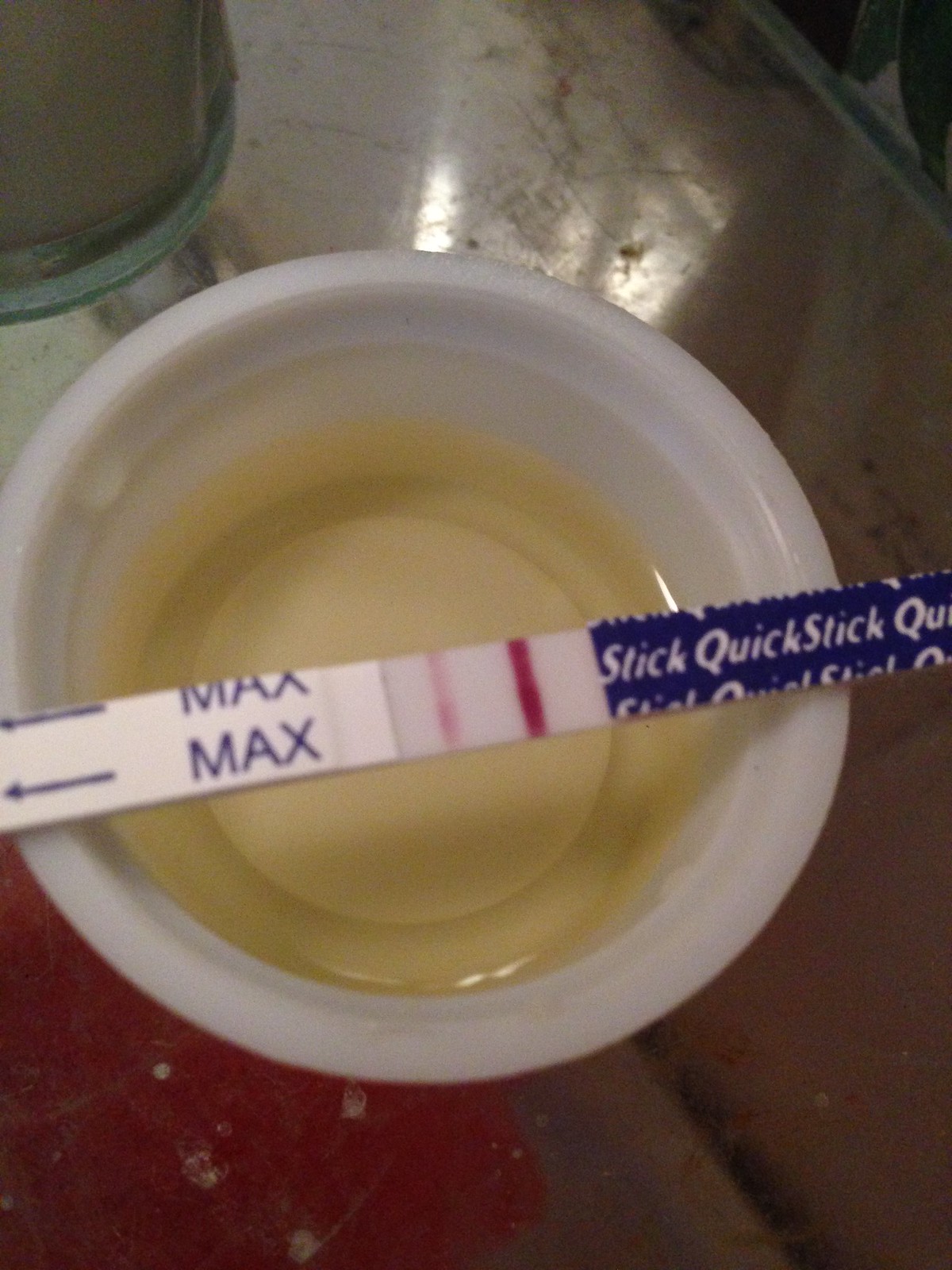The image depicts a white, round specimen cup, viewed from above. The cup is approximately half filled with pale yellow urine. Resting horizontally across the center of the cup is a white dipstick featuring various elements. To the left side of the dipstick, there is purple lettering displaying the word "MAX" in capital letters, accompanied by two arrows pointing left. Moving towards the center, there are two red stripes: a dark red stripe near the center and a fainter red stripe to its left. The right side of the dipstick is purple and repeatedly printed with the phrase "STICK QUICK" in white text.

The specimen cup is placed on a metal countertop. In the lower left corner of the image, a red object is slightly visible, while a pale green object can be seen in the upper left corner, adding subtle color contrasts to the scene.